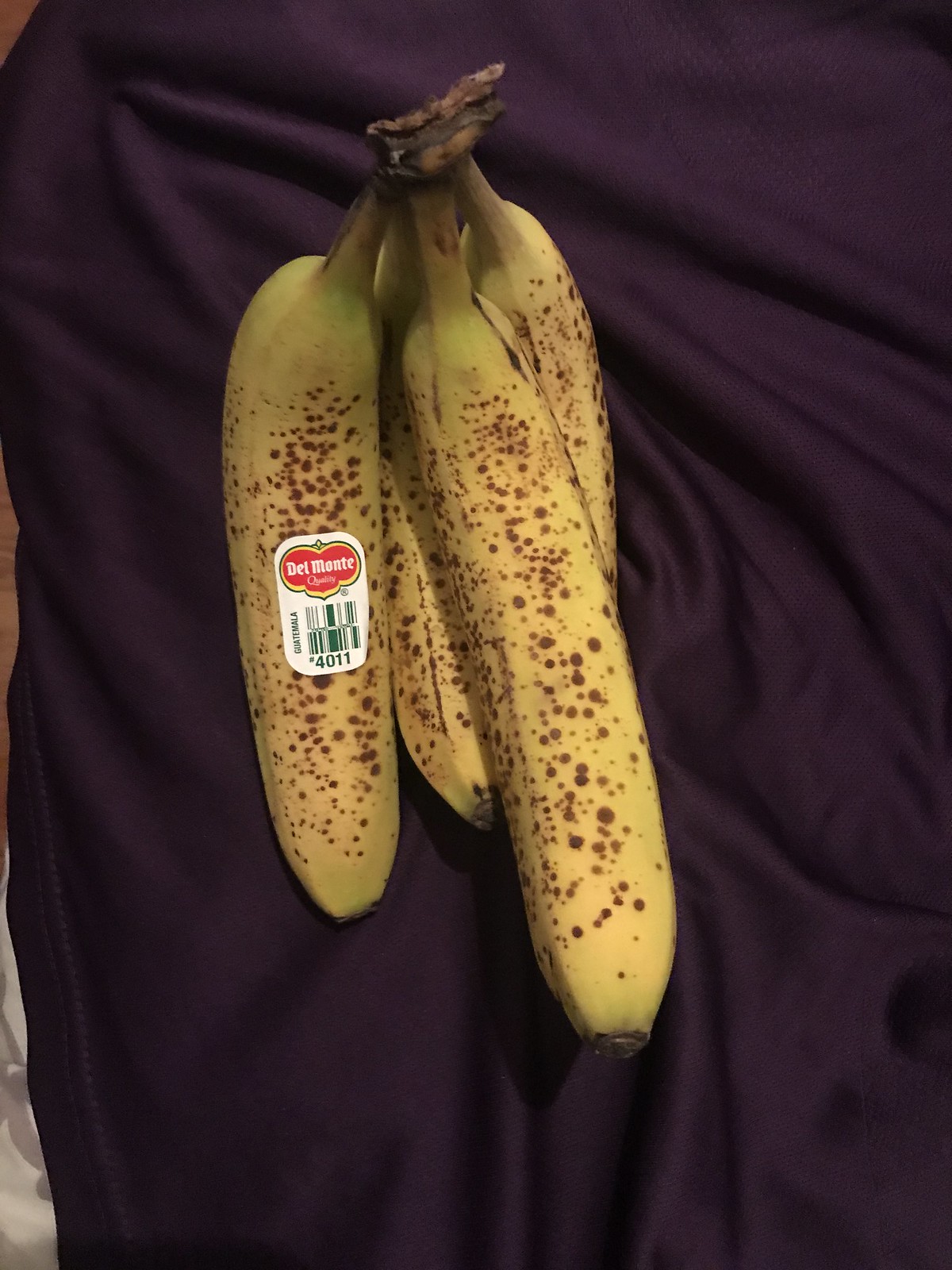This color photograph shows a bunch of four ripe bananas, characterized by their yellow skin dotted with numerous brown spots, suggesting they are at a perfect point for eating. The bananas have a hint of green near the stems and the tips, but are predominantly yellow with a connecting piece that is brown. Notably, the banana on the far left features a prominent Del Monte sticker, which is red with a yellow outline, and includes a barcode and the numbers "4011." The bananas are positioned vertically and rest on a wrinkled piece of plum-colored fabric, with a small section missing in the lower-left corner, revealing a tan surface beneath. The overhead angle of the photograph provides a clear view of the entire bunch set against the dark, textured background.